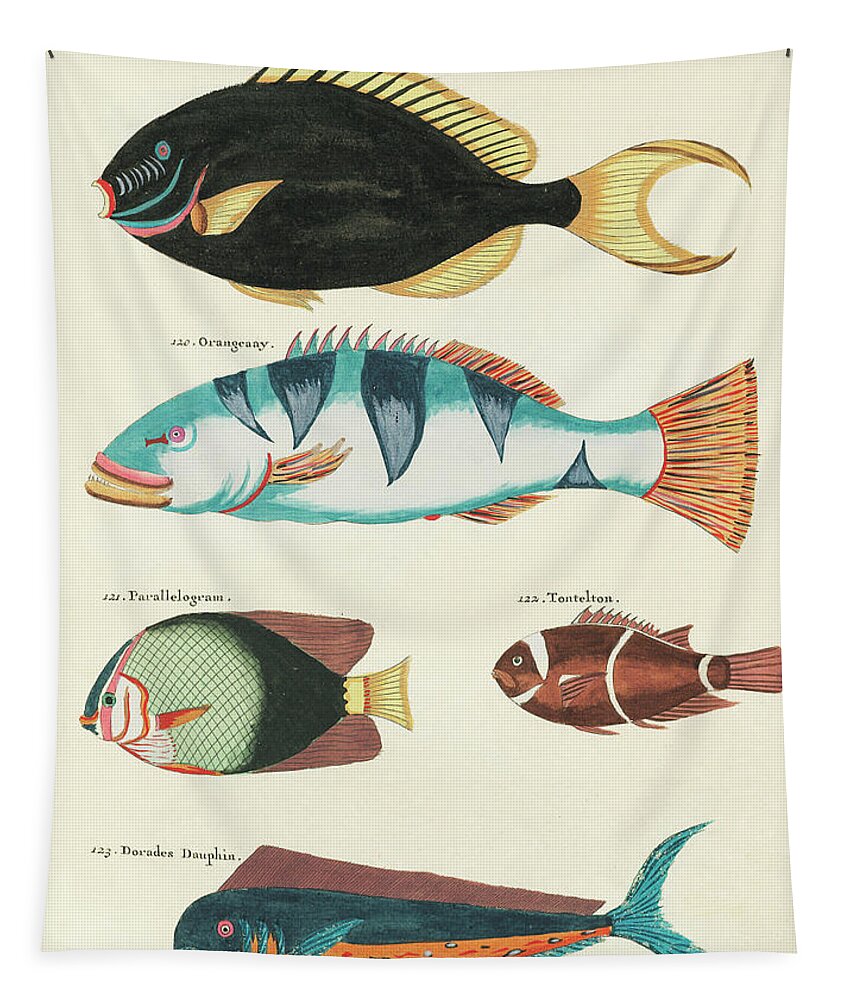The image depicts a color photograph in portrait orientation, showcasing a hand-painted illustration banner of five diverse fish species, each labeled with a title. The canvas cloth, nailed to a surface with black pins at the top, serves as the backdrop. The fish are arranged in a vertical column, all facing left.

At the top of the banner is a black fish with a thick, rounded body shape. It features distinct gold fins and tails, and its face is adorned with pink and blue stripes surrounding its pink and blue eyes. The label of this fish is partially cut off.

The second fish, labeled "120 Orange New York," has a slim turquoise and white body with blue teal markings, orange and turquoise fins, and pink eyes.

The third fish, "121 Parallelogram," is characterized by its two shades of green—light and dark. The light green sections display a plaid pattern with darker green lines, complemented by reddish-brown fins, a yellow tail, and its head exhibiting orange, white, pink, and teal stripes.

The fourth fish, "122 Tontoton," combines blue, brown, and white on its body, with white markings, reddish-brown fins, and a tail.

The final fish at the bottom, labeled "123 Doradis Dauphin" (incorrectly spelled as dolphin), has a teal and orange body with reddish-brown fins, a turquoise tail, and pink eyes.

The fish illustrations, vibrant and varied in color, are painted on a cream-colored fabric digitally printed, suggesting the style of photographic representationalism and realism in color illustrations.